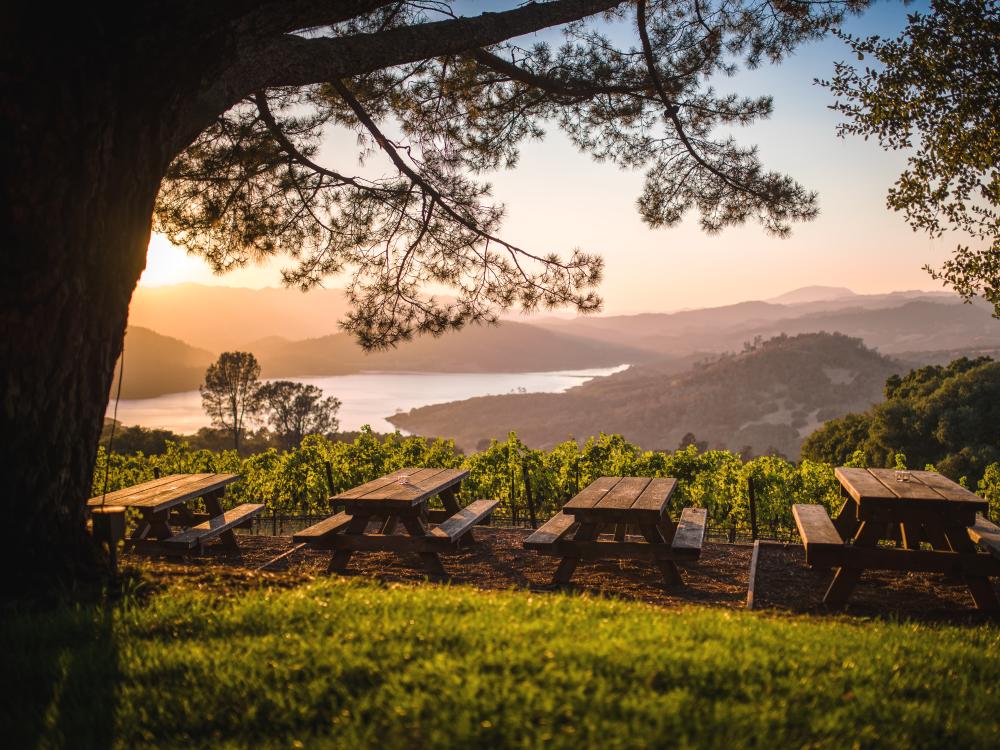In this picturesque landscape photo, we're greeted with a foreground of vibrant green grass leading to a brown, dirt-filled patch hosting four brown wooden picnic tables, some adorned with items. Flanking the right side of the image is a tall tree, with its half-visible trunk framing the photo and branches adorned with pine needles extending over the scene. Beyond the picnic area lies an expanse of green grapevines, hinting at a peaceful winery setting. In the background, a beautiful blue river meanders from the left, framed by rolling hills that gradually ascend to tree-laden mountain ranges. The sky above transitions from a rich, saturated blue at the top to a lighter hue near the horizon. To the left of the image, a golden sun hangs low, suggesting either an early morning rise or a serene evening sunset, illuminating the landscape in a soft, warm glow.